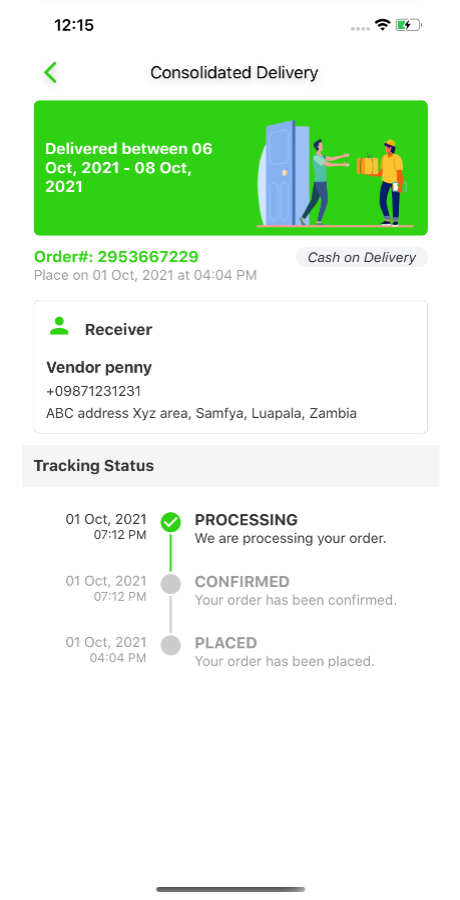The image is an iPhone screenshot displaying an interface that appears to be either an app or a web browser page. The time displayed on the iPhone is 12:15, with no cell service, full Wi-Fi connectivity, and a battery level of less than half charged.

At the top of the screen, there is a green arrow pointing to the left. Below that, the menu bar displays the title "Consolidated Delivery" with a green background. The primary content features two cartoon characters: a man in a green shirt and blue pants stepping out of a blue door, and a woman wearing a yellow hat, yellow shirt, and blue jeans handing him a box. The caption next to this illustration indicates that the delivery occurred between October 6, 2021, and October 8, 2021.

Additional details provided include:
- Order number: 2953667229
- Payment method: Cash on Delivery
- Order placed on: October 1, 2021, at 4:04 PM
- Receiver: Vendor Penny
- Contact number: 09871231231
- Delivery address: ABC Address, XYZ Area, Samfya, Luapula, Zambia

The tracking status history reveals:
1. October 1, 2021, at 7:12 PM – Processing: "We are processing your order."
2. October 1, 2021, at 7:12 PM – Order confirmed.
3. October 1, 2021, at 4:04 PM – Order was placed.

The screenshot clearly depicts an order delivery status for a user located in Zambia, showcasing the journey from order placement to confirmation and processing.